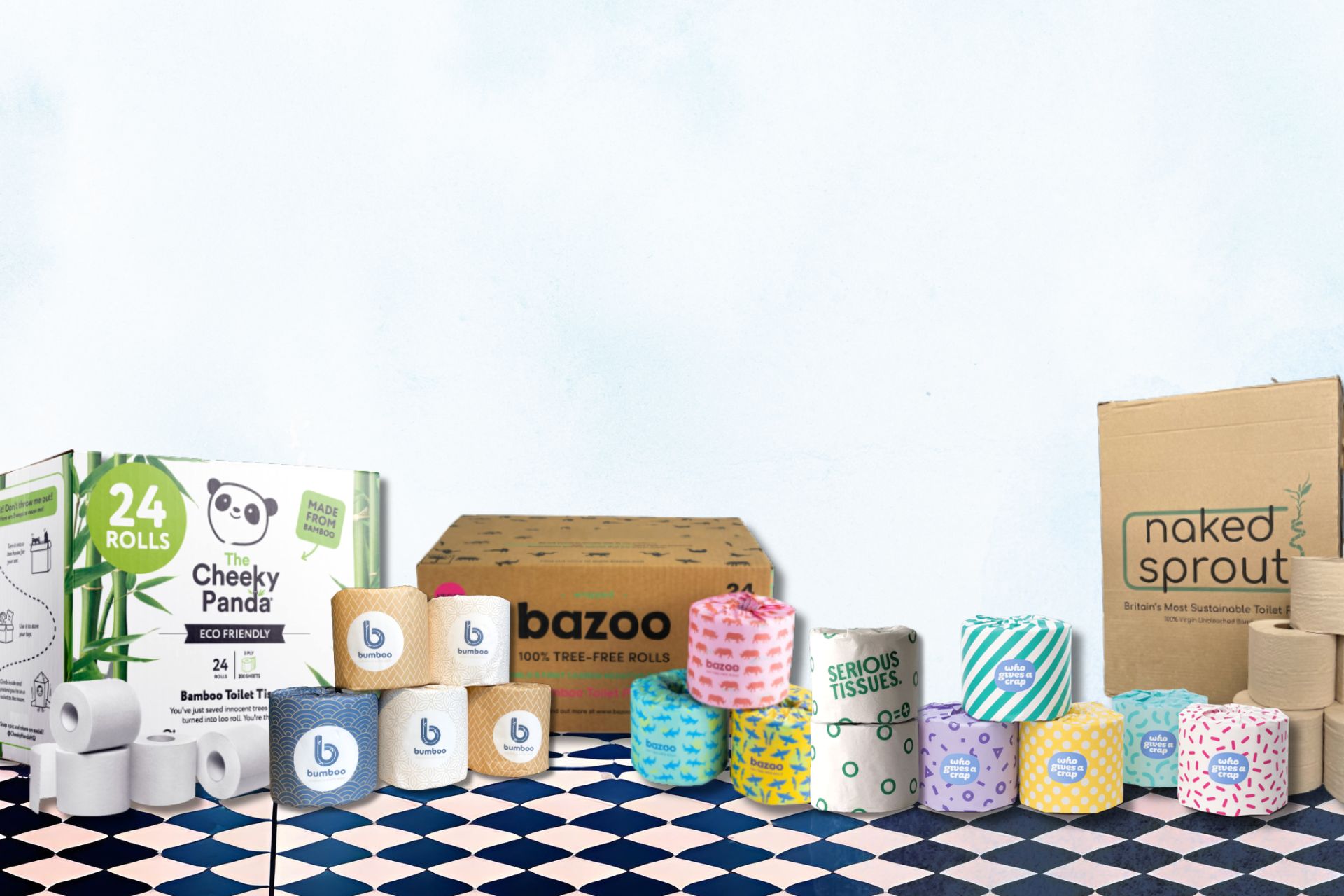The image features a diverse display of toilet paper products arranged on a checkerboard-patterned table with tiles transitioning from black and white to varying shades of blue and white. The lower half of the image is filled with an array of toilet paper rolls and their associated packaging. On the left, there are plain white rolls, and near them is a box labeled "Cheeky Panda" with a green design and an outline of a cartoon panda, advertising 24 eco-friendly rolls. In the middle, a large square cardboard box with black text reads "Bazoo 100% Tree-Free Rolls." The right side features a rectangular box labeled "Naked Sprout" with a green design surrounding the black text. In front of these boxes, various toilet paper rolls are displayed. These include plain brown rolls, a roll with white wrapping and pink accents, a white roll with blue and yellow, another with purple, and others with white and green stripes. Some rolls feature a logo with the letter 'B' and are stacked five high in an arrangement of three rolls on the bottom and two on top. The subtle blue backdrop, which resembles a cloudy sky, adds a soft and calming contrast to the vibrant and varied display of toilet paper below.